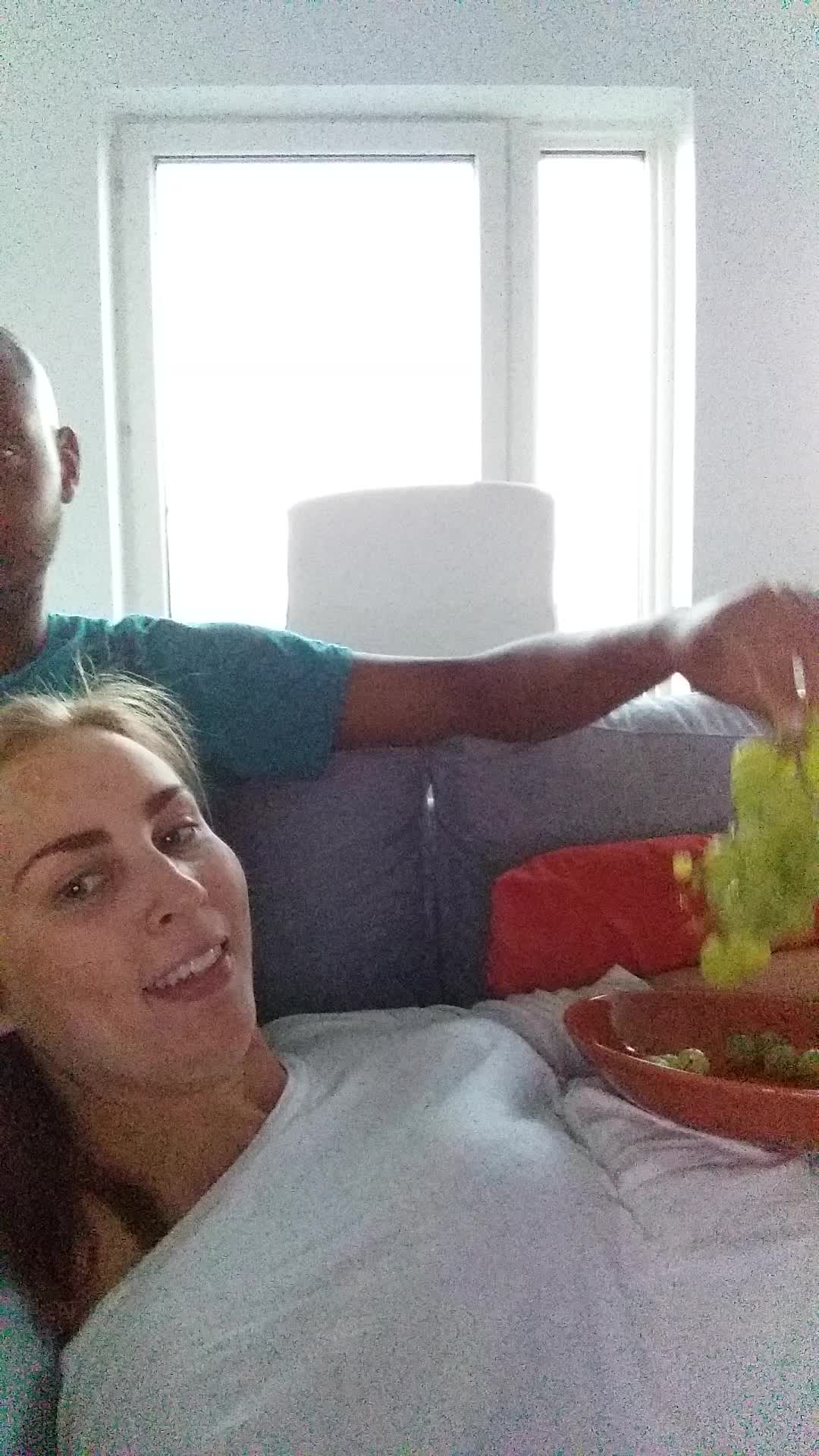This vibrant indoor daytime photograph captures a cozy moment on a light purple, almost gray couch adorned with a red throw pillow. A blonde woman, dressed in a gray t-shirt, reclines on the couch with a red dish of green grapes resting on her chest. She gazes toward the camera, lying slightly inclined with her shoulders and head propped up. Next to her, a gentleman with a shaved head, clad in a blue shirt and blue jeans, sits with his left arm reaching down to pick some grapes from the dish. Although only the left side of his face is visible, he appears to be looking away from the camera. The serene background features a white lamp and a large window that lets in a generous amount of sunlight, softly illuminating the room and enhancing the intimate atmosphere.